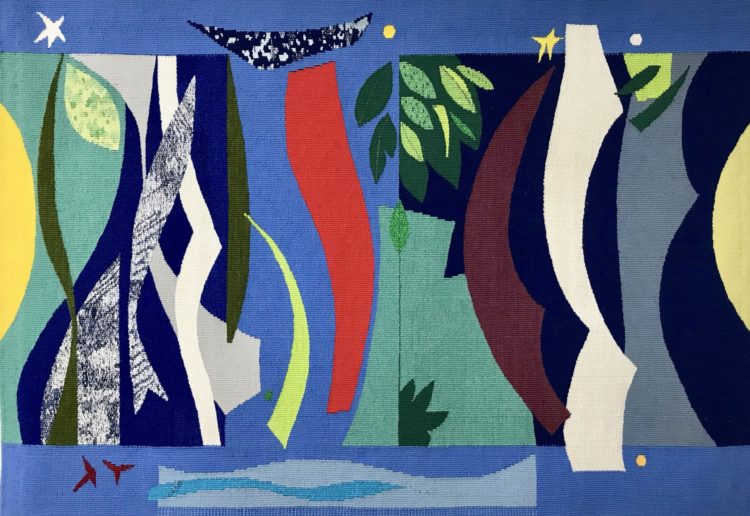This artwork is a vibrant and elaborate fabric collage, showcasing an abstract art style characterized by an array of irregular shapes and colors. The background, composed of blue linen or twill fabric, serves as a canvas for diverse fabric swatches. Predominantly, the colors include light blue, emphasized as a soft backdrop and sky blue accents that give an impression of waves at the bottom of the piece.

The artwork incorporates various long and circular fabric cuttings, layered both vertically and horizontally across the canvas. Central elements include royal and dark blue squares adorned with wavy white abstract shapes. Bright red ribbons, alongside hunter and pea green foliage cut into leaf shapes, add a dynamic dimension to the work. Interspersed within these elements are delicate white and green strands resembling blades of grass. 

Distinctive features include two birds rendered in red near the bottom, and a bush-like shape positioned at the lower part of the composition. Several stars dot the fabric: a white star in the upper left-hand corner and a yellow star on the right side. Additional details such as yellow, white, and orange dots scattered across the artwork, contribute to its playful complexity.

Overall, the piece conveys a rich tapestry of textures and colors, displaying a harmonious yet eclectic mix of fabric swatches meticulously arranged to evoke vibrant and nature-inspired abstract themes.